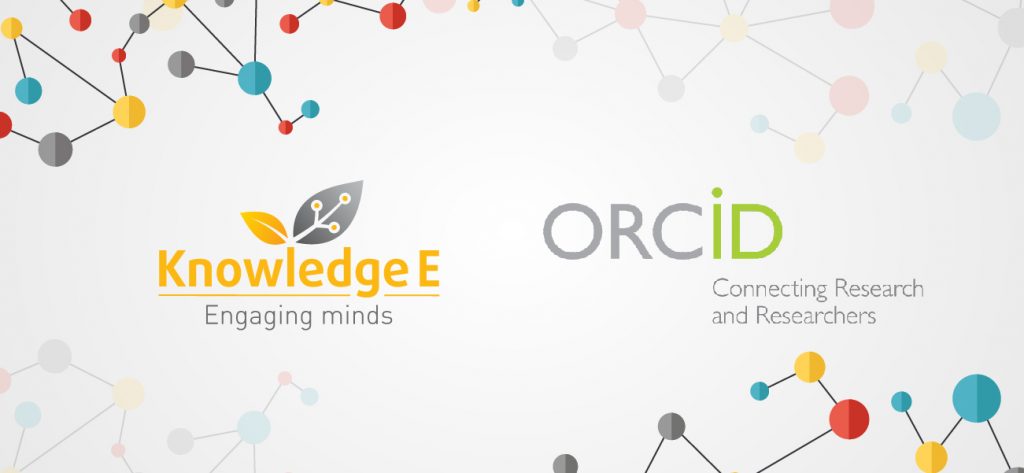The image features the title "Knowledge E" prominently in yellow font. Below the title, the phrase "Engaging Minds" is displayed. Above "Knowledge E," there are two distinct leaves: a smaller orange leaf and a larger black leaf, approximately twice the size of the orange one. The black leaf is intricate, featuring visible veins resembling vines.

In the top left corner of the image, a series of interconnected spheres appear in various colors—gray, blue, and pink—linked by thin lines, forming a web-like pattern. To the right of "Knowledge E," centrally located, the word "ORCID" is visible, with the "ID" portion highlighted in green.

Directly below, starting under the "I" in "ORCID," the text "Connecting Research" is displayed over two lines. Beneath this text, there is a repeated graphic of interconnected, multi-colored dots, mirroring the pattern in the top left corner.

In the top right and bottom left corners of the image, faint, mirrored versions of the interconnected spheres and lines appear, adding symmetry to the design. The background is a light gray color, and the connecting lines throughout the image resemble taut black strings, enhancing the neat, organized aesthetic.